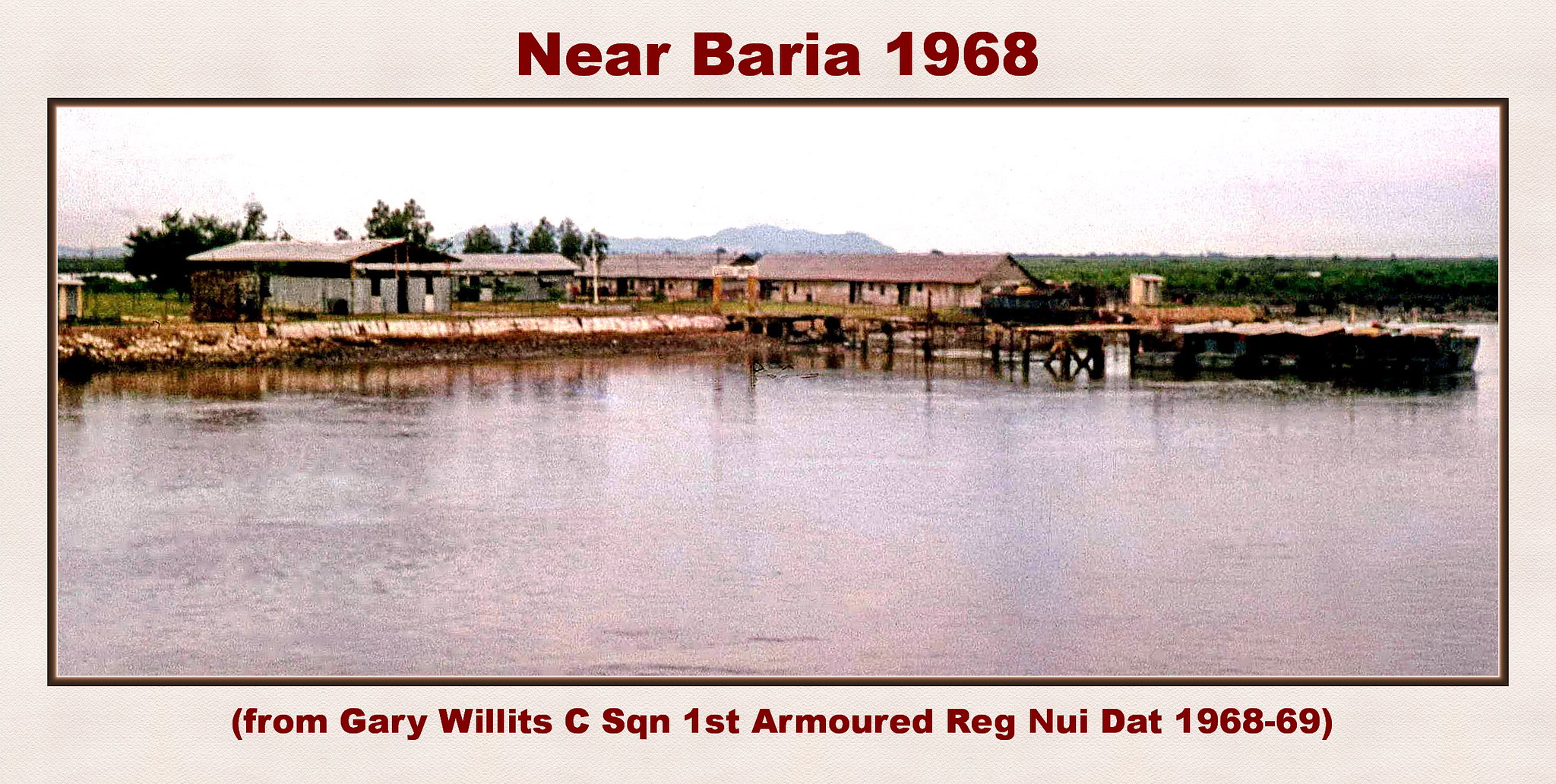This is a grainy, slightly blurry photograph capturing a scene from Vietnam in 1968. The image features a tranquil body of water in the foreground, with uneven, rickety docks extending into it. In the background, there are low-level, rough building structures characteristic of a remote village. Faintly visible behind the structures are tropical fields and hills or mountains. A flag can be seen, with a few indistinct figures nearby. Notable text in red at the top of the image reads, "Near Baria, 1968," while the bottom text in parentheses states, "From Gary Willetts, C-Squadron, 1st Armoured Regiment, Nui Dat, 1968-69."